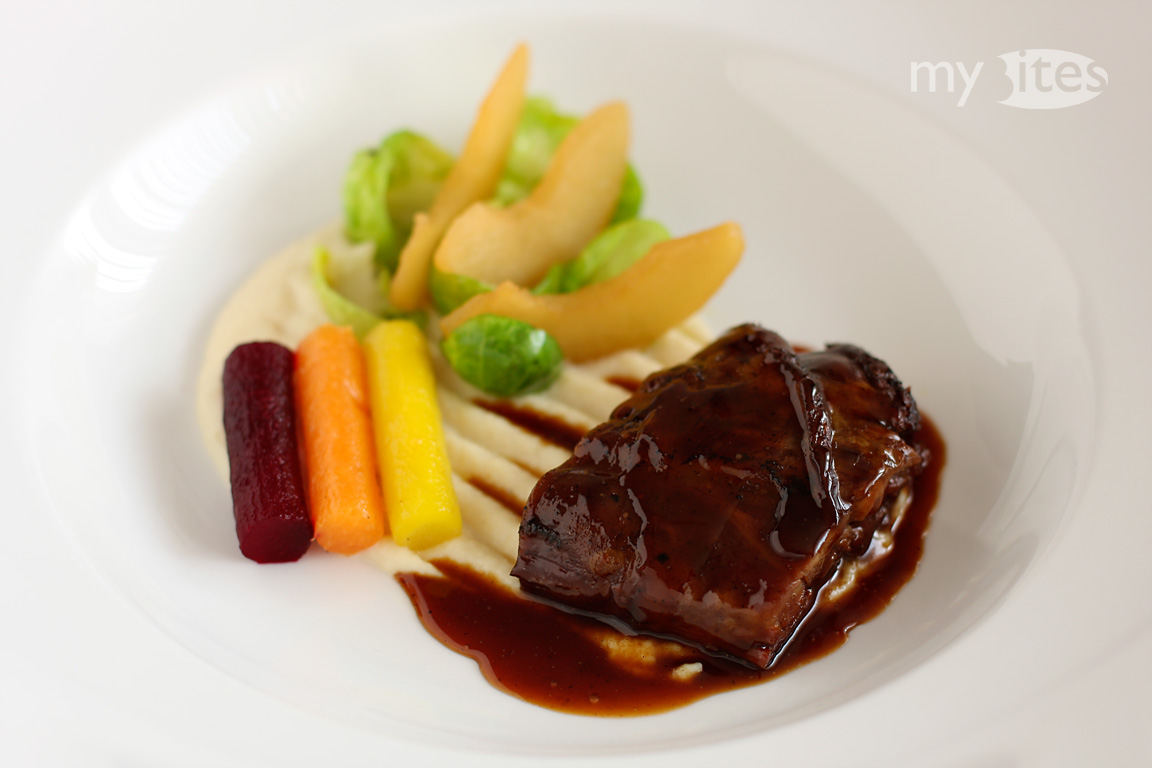This photo features a meticulously plated dinner entree on a slightly indented, white plate. At the center is a small, roasted beef piece, generously draped in dark gravy, served atop a bed of creamy mashed potatoes. To the left of the beef, three perfectly cut baby carrots—one dark purple, one orange, and one yellow—add a colorful touch. Adjacent to the carrots are wedges of a pale, whitish-yellow fruit, likely pear, resting on a small bed of Brussels sprout leaves. The detailed composition and vibrant color contrast of the various elements make for an appealing and appetizing presentation.